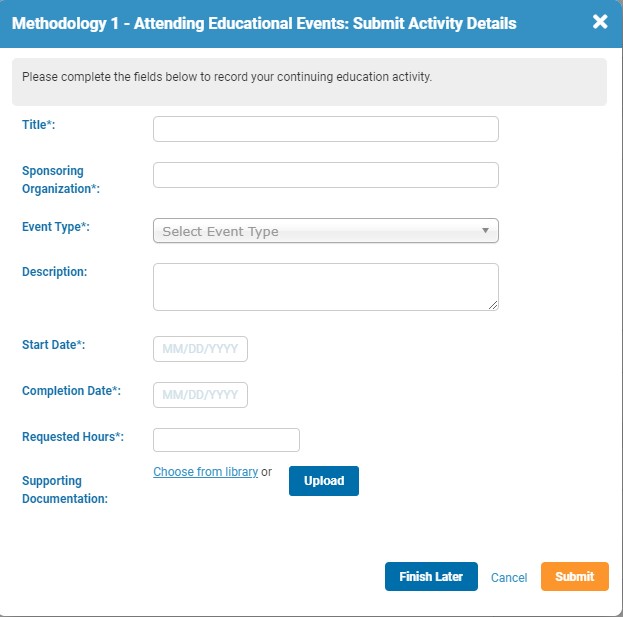In the image, there is an interface resembling a form for enrolling in a school class, specifically titled "Mythology 1 - Attending Educational Events." The top of the form features a long blue rectangle with the title in white lettering and a white 'X' icon on the right side, likely for closing the form.

Directly below, a light gray box contains a prompt in black lettering: "Please complete the fields below to record your continuing education activity." Following this, several fields are presented for user input:

1. **Title:** Indicated by an asterisk, with a white text box for entering the title of the activity.
2. **Sponsoring Organization:** Also marked with an asterisk, this field includes another text box for the name of the sponsoring organization.
3. **Event Type:** Accompanied by an asterisk, with a dropdown menu that defaults to "Select event type" in gray lettering.

Below these fields, there is a **Description** box for adding detailed information about the event. 

The **Start Date** field, marked with an asterisk, requires input in the format of two-month, two-day, and four-digit year. Similarly, a **Completion Date** field, using the same date format, is provided.

Further down, there is a section for **Requested Hours**, allowing users to input the number of hours being requested. 

For **Supporting Documentation**, users are prompted in blue lettering to "Choose from library or upload," with an adjacent blue button labeled "Upload" in white text.

At the bottom of the form, there are three buttons for submission control:
- A blue "Finish Later" button with white lettering.
- A white "Cancel" button with blue lettering.
- An orange "Submit" button with white lettering.

The entire form is clearly structured, guiding the user through the process of recording their educational activity details.